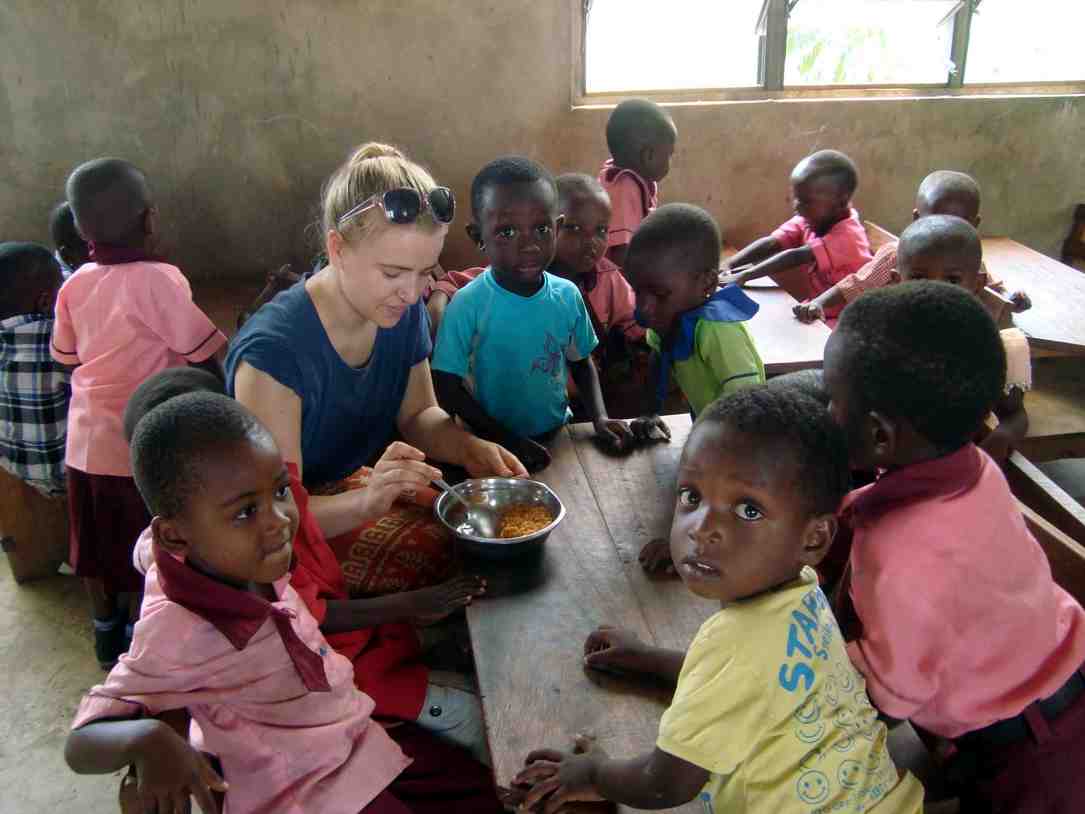In an indoor setting, likely in Africa, a group of young children, around the ages of four to six, are seated at light wooden picnic tables on a concrete floor, surrounded by dark gray walls with windows letting in ample daylight. A white woman with dirty blonde hair tied back in a bun, wearing a blue shirt with sunglasses perched on her head, sits among them. She has a red cloth over her lap and appears to be feeding the children from a stainless steel bowl with a spoon, possibly serving rice. The children, who are black, are dressed in various brightly colored shirts—yellow, pink, blue, green, and checkered black and white. One boy in a yellow shirt and another in a pink shirt are looking directly at the camera, while others focus on the woman or the bowl of food. The scene conveys a moment of care and nourishment in this communal setting.